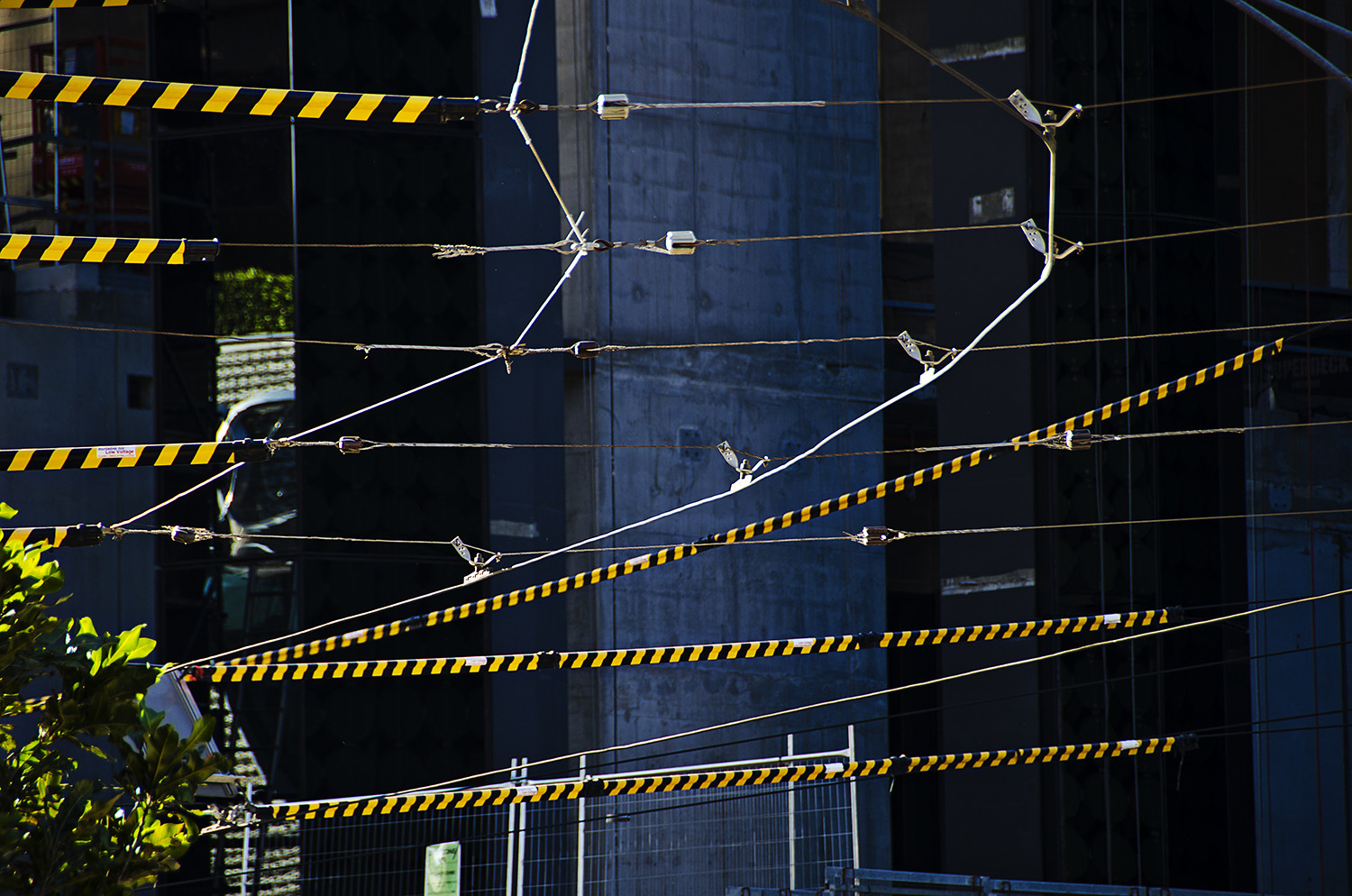This horizontally aligned rectangular photograph, set outdoors in a city during the day, prominently features a catenary system for mass transit. Dominating the scene are two parallel sets of thin, round wires, interlaced with additional supporting wires. These supporting wires are distinctively marked with alternating black and yellow diagonal bands. Appearing sporadically on the wires, extending both horizontally and upward, are lengthening branches equipped with small clips.

In the lower left-hand corner of the image, a cluster of trees backlit by the sun reveals bright green and dark green leaves. Adjacent to the trees, partially legible text is scribbled but remains unreadable. A green sign on a fence in the foreground can be seen, with the visible word "day" amid otherwise indiscernible writing.

In the background, a tall concrete structure extends vertically, characterized by its dark gray, slightly blue-tinted stone wall. The photo captures a cement pillar that could be part of a building, establishing an urban environment. The overall composition blends elements of nature and urban infrastructure, showcasing the intricate network of the catenary system under a city sky.